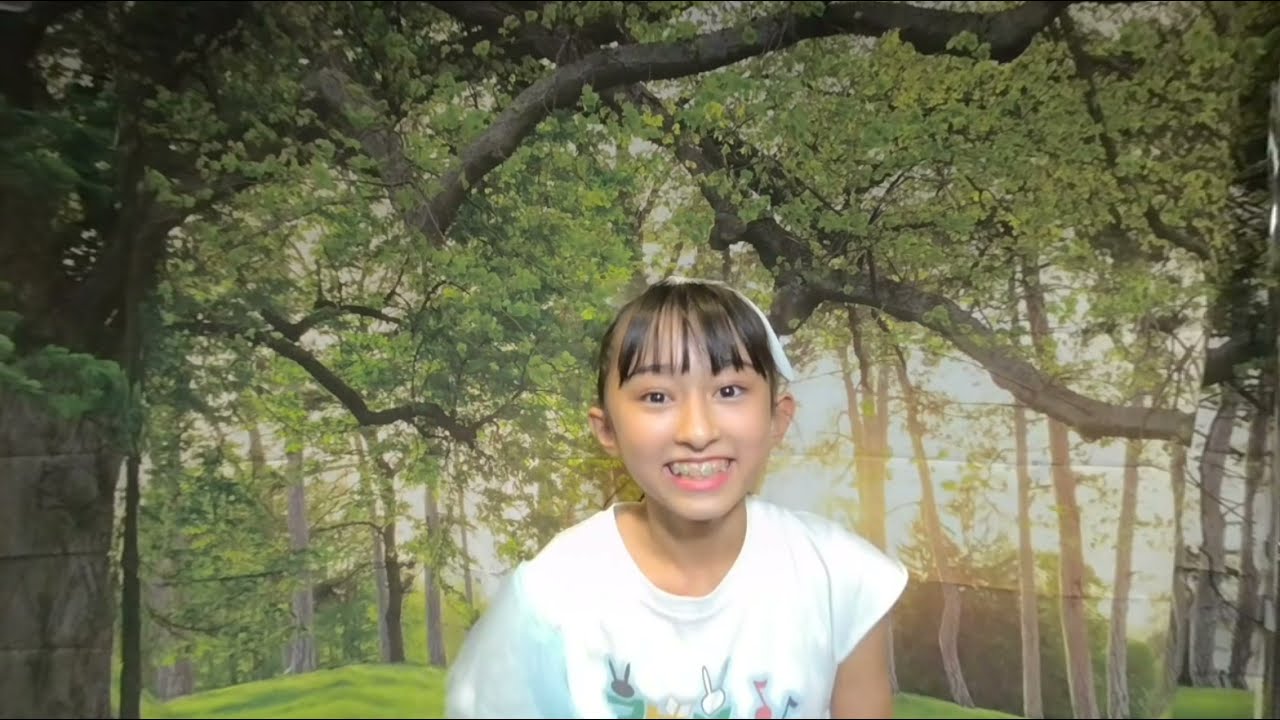A young girl, approximately 10 or 11 years old, stands smiling directly into the camera, her expression revealing braces on her teeth. She has black hair with bangs, tied back, and adorned with a light blue ribbon or bow. Her brown eyes and joyful smile complement her outfit—a short-sleeved white shirt decorated with a pattern of music notes. The background features an indoor setting designed to mimic an outdoor environment with numerous trees, branches, and leaves, though the setting appears artificial, possibly a backdrop with visible folds and lines. Despite the indoor setting, sunlight filters through, adding a realistic touch to the scene. Some stone elements are visible in the bottom left corner.